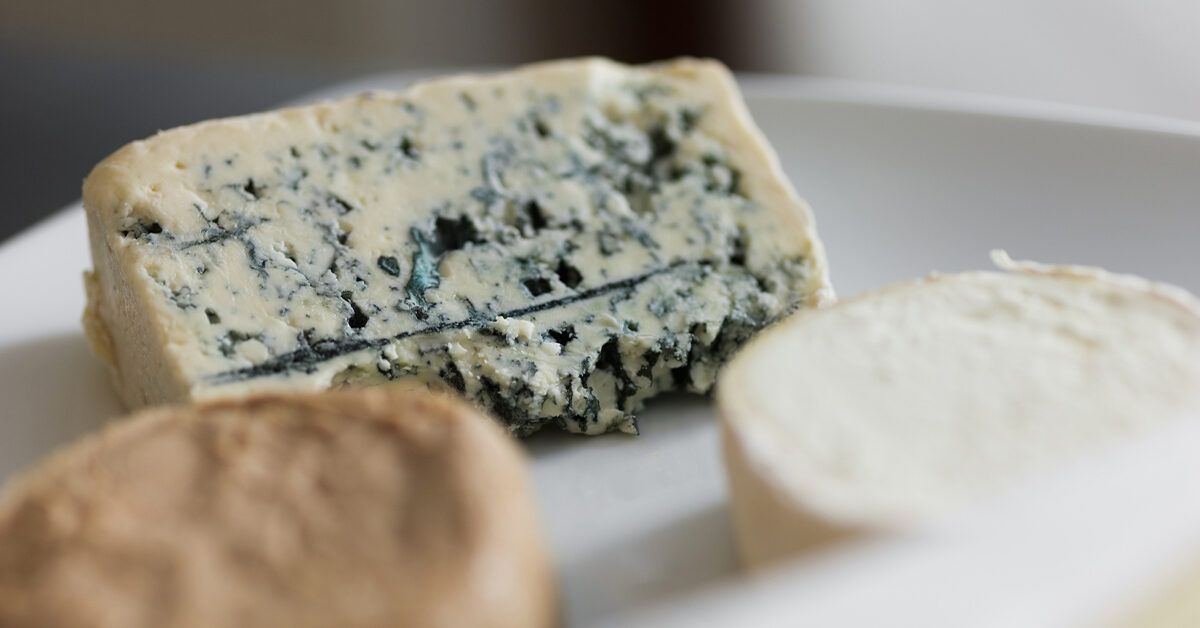The image showcases a professionally captured close-up of a white plate displaying three distinct pieces of what appears to be cheese. The two front pieces are circular and slightly blurred, one darker and the other ivory-colored, about an inch high, possibly a roll or a wedge of cheese. Both are out of focus to draw attention to the item in the background. This focused item is a rectangular piece of cheese, pale yellow with dark specks, resembling a half-eaten blue cheese. The photo is lit from the right, creating subtle shadows cast from right to left. This elegant and simple arrangement likely suggests the setting of an upscale restaurant, with the intent of showcasing the cheeses, perhaps for an advertisement or a website. The overall ambiance is sophisticated, with a minimalistic background that keeps the viewer's focus on the cheese presentation.